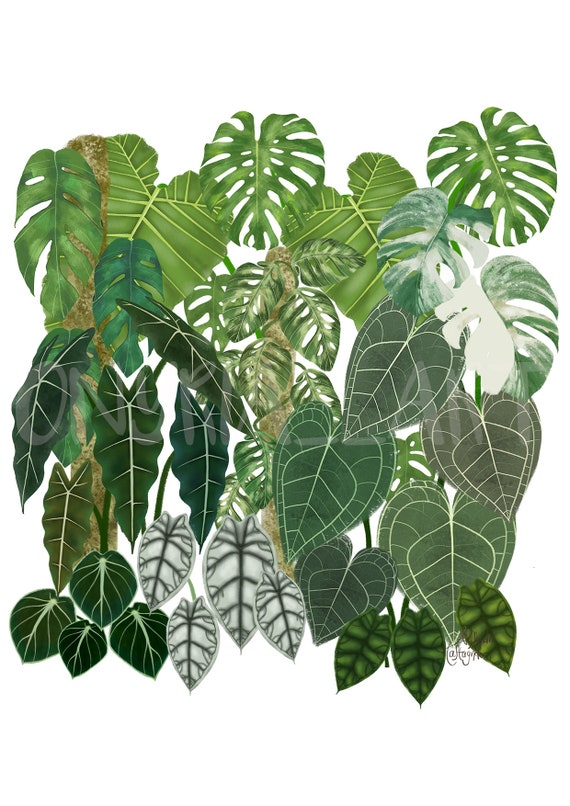The image is a highly detailed digital artwork showcasing a variety of large leaves that bear a striking resemblance to palm leaves. Each leaf is distinct yet shares common features such as elongated, oval shapes with prominent central veins. One notable type is the elephant ear leaf, which possesses an almost heart-shaped form with thin, strip-like cutouts and small holes, rendered in a medium green hue. Among these, genuine heart-shaped leaves are visible, especially along the top row. There's a brown, stick-like element on the right and in the middle, appearing like metal posts adorned with the same perforated leaves. Heart-shaped leaves on the bottom right exhibit green coloration accentuated by white veins, whereas leaves on the left are darker and slightly thinner. The overall palette ranges from dark to light green, with some leaves near the bottom displaying yellow accents or even a blend of white and black veins. The bright, clear setting enhances the detailed depiction. A faint watermark at the bottom right corner is barely legible, possibly reading "onee play." The image's realistic coloring and shading blur the line between actual photographs and digital drawings, particularly noticeable in different parts of the artwork.